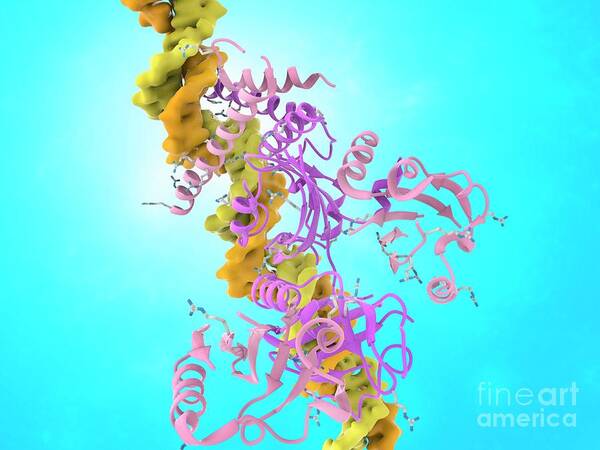This digital image features a bright turquoise-blue background that gradually lightens around the middle, creating a delicate highlight. Dominating the image is a cascade of colorful, spiraled coils reminiscent of party streamers, arranged in a vertical diagonal line that stretches from the top-left to the bottom-right third of the frame. The coils are interwoven and interspersed in vibrant hues of pink, purple, green, orange, and yellow, with some tightly wound together and others dangling loosely, akin to the branches of a festive tree. In the lower right corner, a faint, translucent inscription reads "Fine Art America," adding a subtle celebratory touch to this visually dynamic composition.